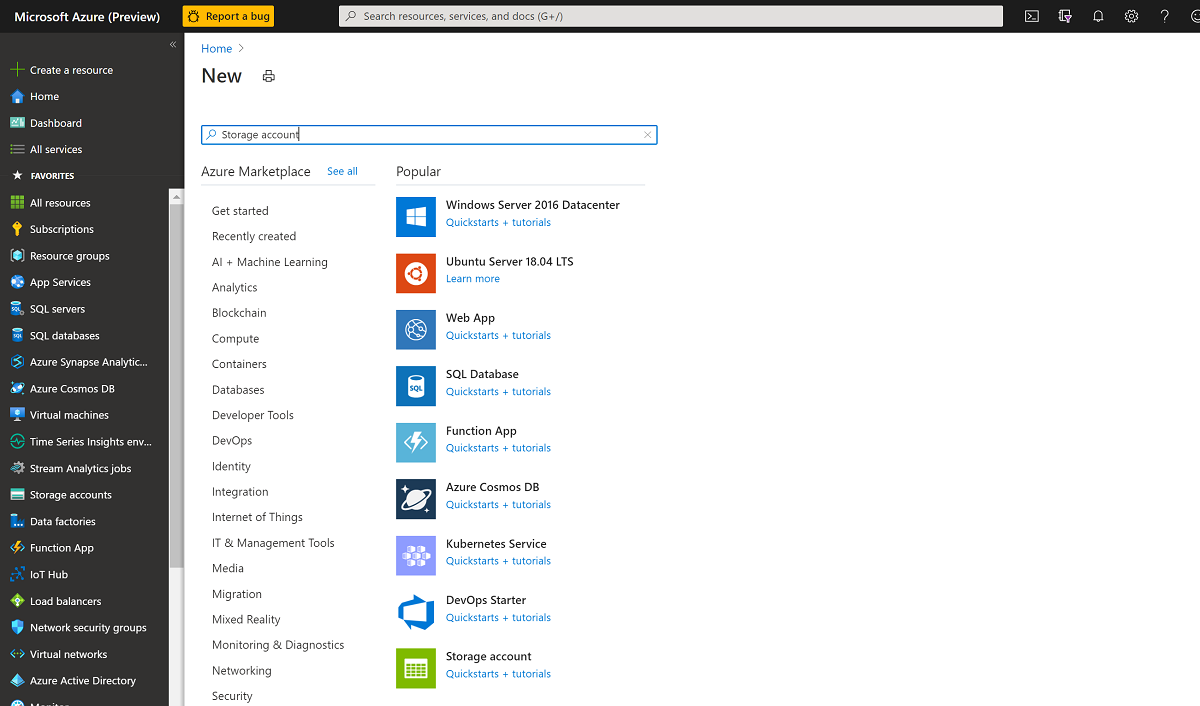This screenshot showcases the homepage of an individual's personal Microsoft Azure account, currently set to a black and white theme. The user has entered "storage account" into the search bar, yielding a selection of diverse options. Prominent among these options are Windows Server 2016 Datacenter, Ubuntu Server 18.04 LTS, web app, SQL database, and DevOps starter. The interface also highlights popular choices for IT management tools, networking, safety features, and bug reporting. Additionally, there are integration possibilities for AI and machine learning technologies. The left-hand column of the screen features numerous other options for navigation and account management.